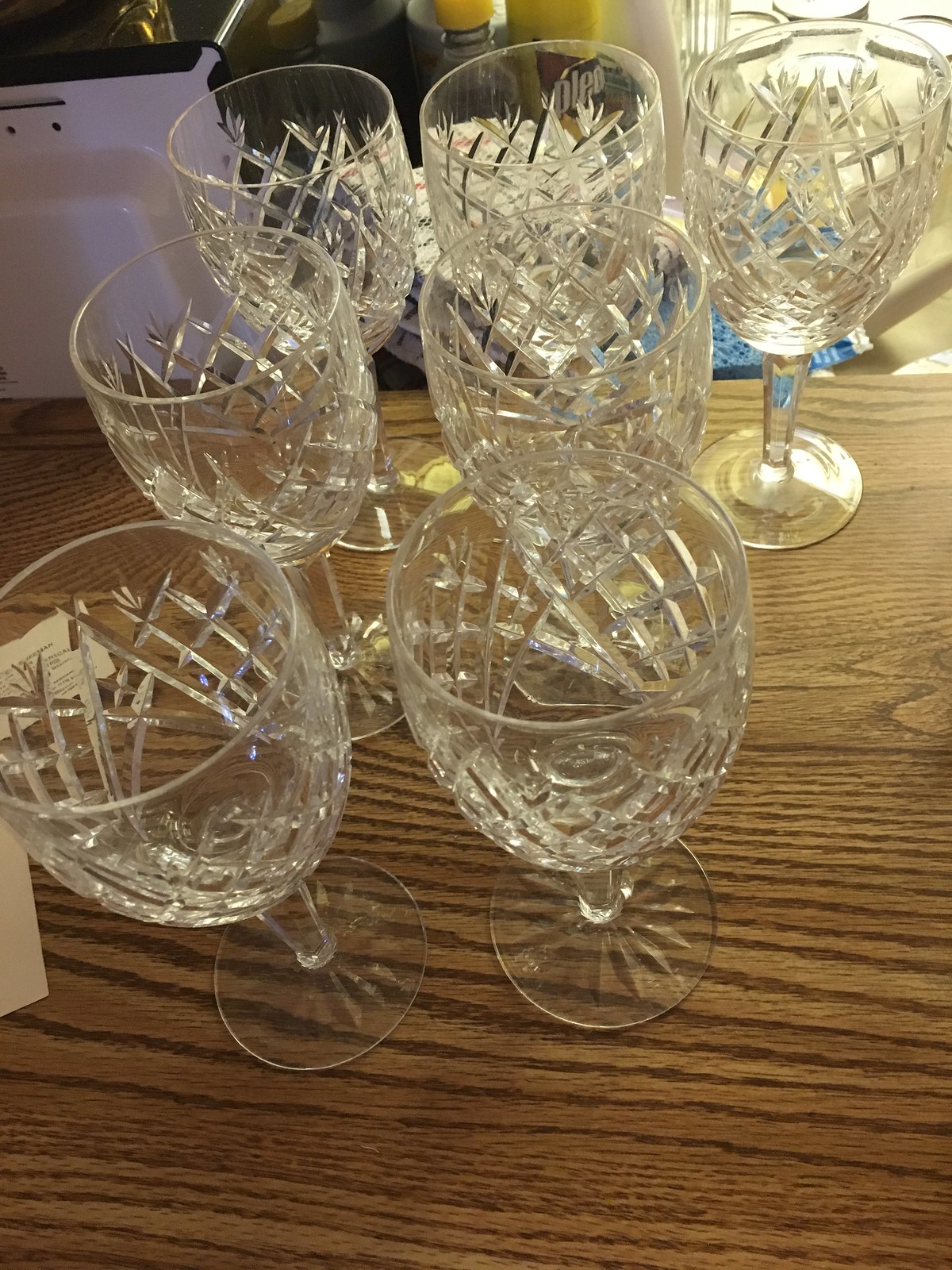In an interior setting, a photograph captures seven identical cut crystal goblets arranged on a light brown oak woodgrain table. The goblets, standing upright with their long stems and round bases, exhibit intricate criss-cross patterns etched into the crystal exterior. The light streaming in from a nearby window illuminates the scene from the top right, casting a gentle glow on the glasses. Positioned in a formation of two in the front, two in the middle, and three in the back, these empty goblets seem to have been recently cleaned, awaiting storage. Behind the table, a partially visible microwave oven with a white body and black top can be discerned, alongside cleaning products, possibly a spray can of Pledge and other indistinguishable items. Despite the casual nature of the photo, it highlights the delicate craftsmanship of the goblets amidst a domestic backdrop.